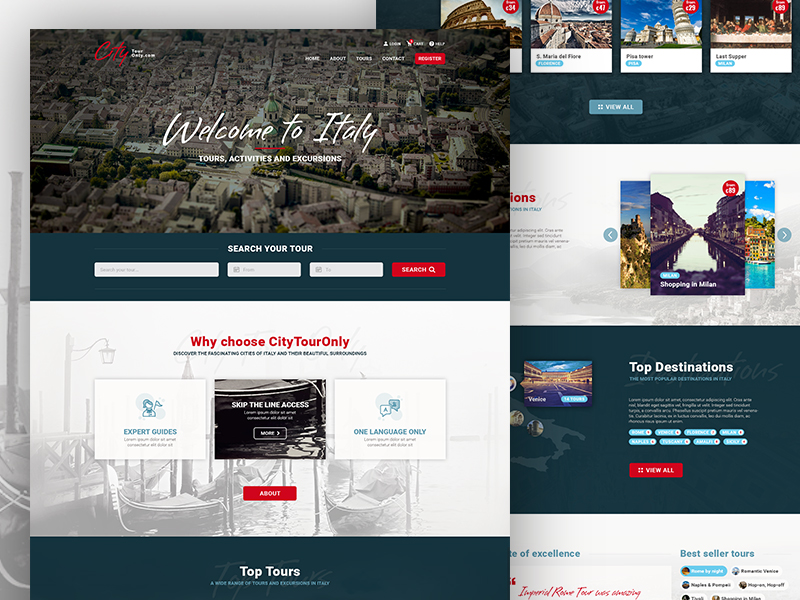The image showcases a sprawling cityscape adorned with numerous stone buildings, predominantly in light brown hues. Interspersed among the urban expanse are dense patches of trees, creating a harmonious blend of nature and architecture. The focal point remains the vast city.

In the upper left corner, the word "city" is prominently displayed in red text. Central to the image is a white, cursive text warmly greeting viewers with "Welcome to Italy," underlined in red for emphasis. Below this, the phrases "tours, activities, and excursions" as well as "search your tour" are shown. Accompanying these instructions are three white rectangles and a conspicuous red rectangle on the right side, emblazoned with the word "search."

Beneath this, in red text, a question reads, "Why choose city tour only?" The provided options are summarized with accompanying visuals: "Expert guides," "Skip the line access" illustrated by an image of a boat near water, and "One language only." Further to the right, a smaller rectangle labeled "about" offers more information. Adjacent to this, a picturesque scene displays buildings flanking a water canal, captioned "Shopping in Milan."

Towards the bottom right, under the heading "Top Destinations," are eight small blue rectangles, each representing different locations. Concluding the array of information is a small red rectangle with the phrase "view all" inside, encouraging exploration of additional destinations.